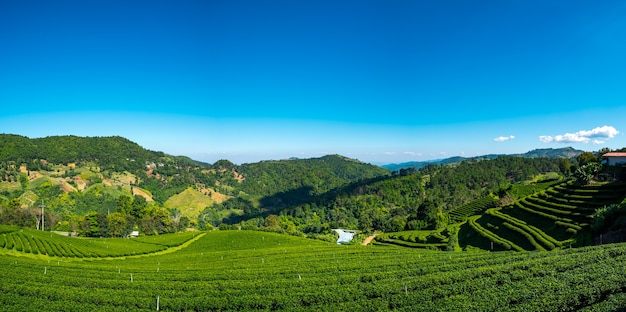This daytime outdoor photograph captures a terraced agricultural landscape viewed from the top of a hill. The rectangular image, approximately four inches wide by two inches high, showcases a series of methodically arranged horizontal rows of green-topped crops cascading down the hillside. These terraces stretch out to the left and right, framed by undulating hillsides that also feature layered cultivation. At the center right of the image, a white house with a red slanted roof provides a focal point amidst the greenery. Beyond the cultivated fields, the landscape rises into a backdrop of dense natural foliage, consisting of vibrant green bushes and trees. The upper half of the photograph features a clear blue sky with a slight white haze along the horizon and some wispy white clouds towards the right side, completing the picturesque and serene rural scene.